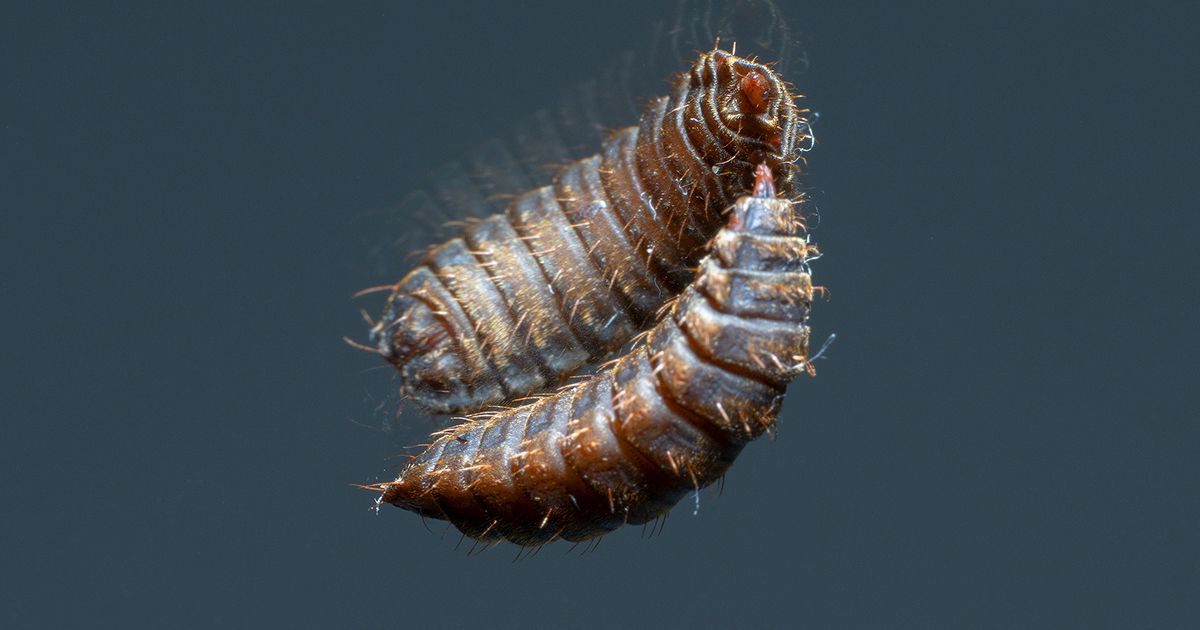This image features an extreme close-up of a single segmented insect, likely a larva, reflected on a mirrored surface. The larva has a chitinous exoskeleton that gradates from brown to amber, with sparse, spike-like hairs protruding from each segment. The body of the insect is curled in a crescent shape, and a distinct reddish or pinkish proboscis-like appendage extends from its front. The background is a slate blue or grayish-blue, creating a stark contrast that highlights the intricate textures and details of the larva, including the underside visible in the reflection. The absence of limbs and the floating appearance, potentially from being photographed through glass, adds to the enigmatic, almost ethereal quality of the scene.